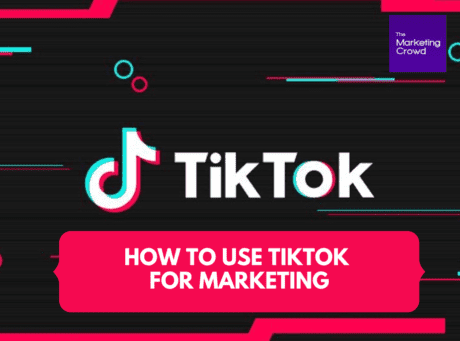This screen capture likely depicts an advertisement for a marketing event or tutorial on utilizing TikTok for marketing purposes. The background is primarily black with several colorful accents and shapes creating a dynamic visual layout. 

At the top of the image, a pink line stretches across, followed by another parallel pink line. Just below these lines, a purple square contains the text "The Marketing Crowd" written in bold white letters. Adjacent to this square is a teal circle, adding to the colorful composition. 

Beneath, a mix of teal and pink lines intersects the design, leading to a section on the opposite side where a teal circle and a pink circle are featured. Further down, the word "TikTok" is displayed prominently. The 'O' in "TikTok" is uniquely stylized with teal and pink shadows, giving it a whimsical and eye-catching appearance. 

Below the "TikTok" text, a bold pink rectangle stands out with the white text "How to Use TikTok for Marketing," ensuring the message is easy to read and attention-grabbing. A pink line and a small teal dot follow this, adding further accents to the design.

The bottom of the image features a pink shape resembling a lightning bolt, also in a bold and easy-to-read font. The overall design is vibrant with a playful use of colors and shapes, effectively emphasizing the text and drawing the viewer's attention to the key message.